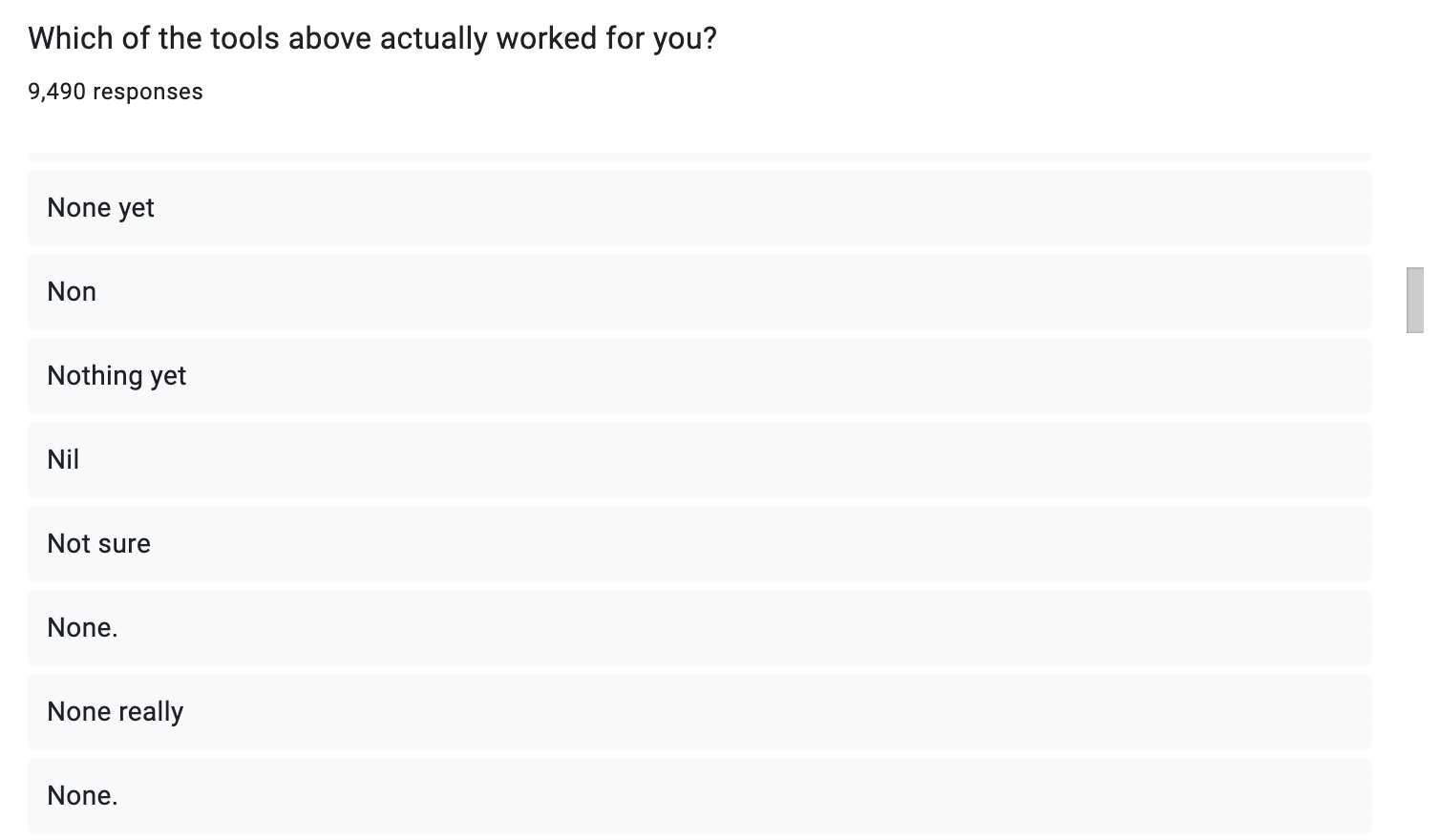This image is a screenshot of a survey or form that has collected users' responses to the question, "Which of the tools above actually worked for you?" displayed prominently at the top. Below this question, it is noted that there have been 9,490 responses. The responses are displayed in a vertical list of light gray text boxes with black text, each separated by a white line. The top response reads "None yet," followed by a series of similar replies: "None," "Nothing yet," "Nil," "Not sure," "None." (with a period), "None really," and another "None." (with a period). A small gray vertical rectangle, likely the scroll bar for the form or website, is visible next to the second text box. The first word in each response is capitalized, while any subsequent words are not. At the top of the list, there is a subtle gray line indicating a possible cutoff text box or a division between the question and the response list.